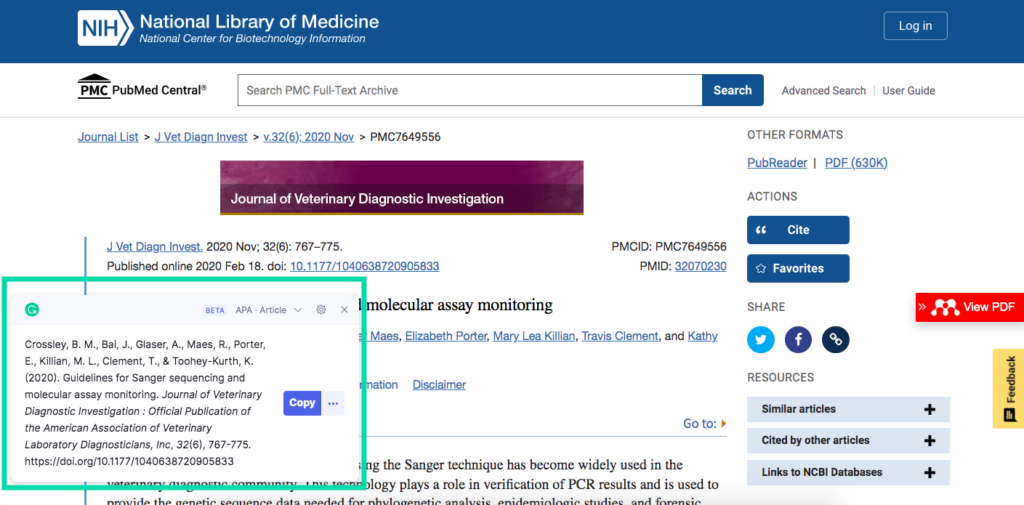This image depicts a webpage from the National Library of Medicine's National Center for Biotechnology Information (NCBI) site, specifically within the PMC (PubMed Central) database. At the top, there is a prominent search bar and options to log in. Below, the page features a specific journal entry from the "Journal of Veterinary Diagnostic Investigation," with publication details noting it was first published online on February 18, 2020, with a November 2020 issue date.

A pop-up box highlights the "Official Publication of the American Association of Veterinary Laboratory Diagnosticians Inc.," detailing guidelines for Sanger Sequencing Molecule Assay Monitoring. Unfortunately, a large portion of the text is cut off, rendering it unreadable in the image.

On the right-hand side, the page offers various access options including PubReader, PDF, and tools for actions like citing or adding the article to favorites. There are social media share links for Twitter, Facebook, and another unspecified platform. Additionally, there are sections for similar articles, citations by other works, and links to related resources within the NCBI database.